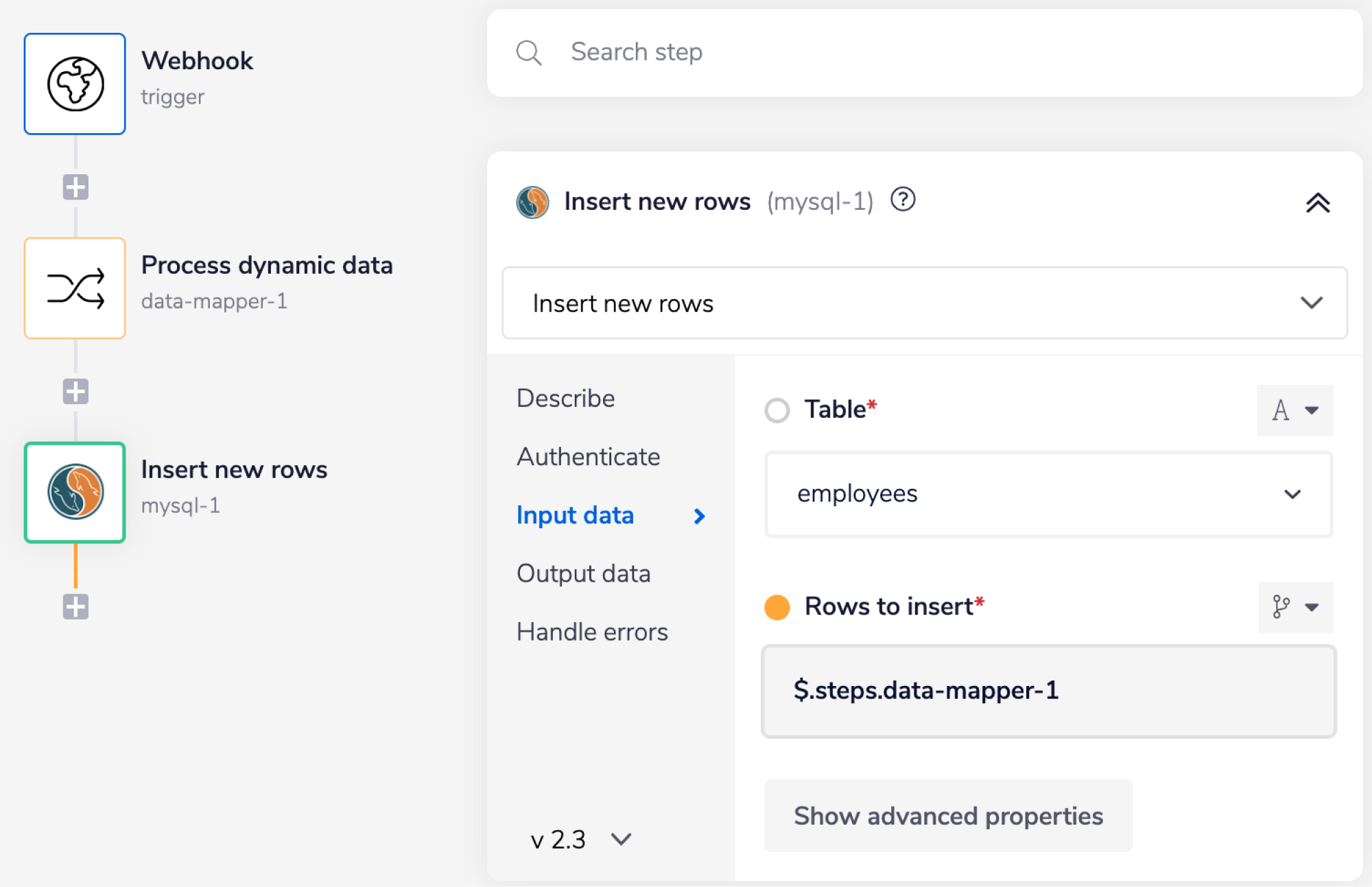The image depicts a section of a technical interface, presumably part of a larger application. On the left, there are three modules labeled "Webhook," "Process Dynamic Data," and "Insert New Rows," suggesting a sequential workflow. Above these modules, a search bar is prominently placed. To the right, a detailed pane provides further functionality and options. Under the "Insert New Rows" module, it's specified to use MySQL, indicating database operations. The interface implies that a table already exists and is undergoing modifications to insert additional rows, with specific data points chosen for insertion. There is an advanced properties button for more detailed configurations. The bottom of the window displays the version number, v2.3. This setup suggests a sophisticated interface for handling large-scale data operations and interactions, possibly related to networking or internet applications.